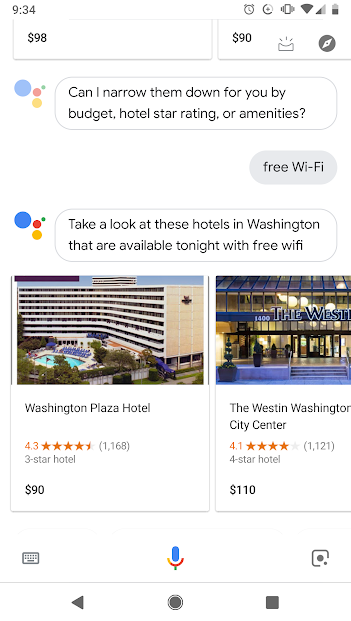The image is a screenshot taken from a smartphone. In the top left corner, the screen displays a balance of $9.34. On the top right corner, several icons are visible, including an alarm, Wi-Fi signal, cellular signal strength, and battery status. Directly below, there are two boxes: the left one showing $98 and the right one showing $90 with two unrecognizable icons inside.

The main section of the screenshot features a conversation with a white background. The individual's profile picture appears on the left, designed with a large blue circle and a smaller red circle positioned to the right, with an even smaller orange circle beneath it. In the central conversation area, a text box from the profile picture says, "Can I narrow them down for you by budget, hotel star rating, or amenities?" In response, a dark grey text box underneath states "free wifi."

Further down in the conversation, the same profile picture text box suggests, "Take a look at these hotels in Washington that are available tonight with free wifi." Following this message, the screen lists two hotel options: the Washington Plaza Hotel and the Westin Washington City Center.